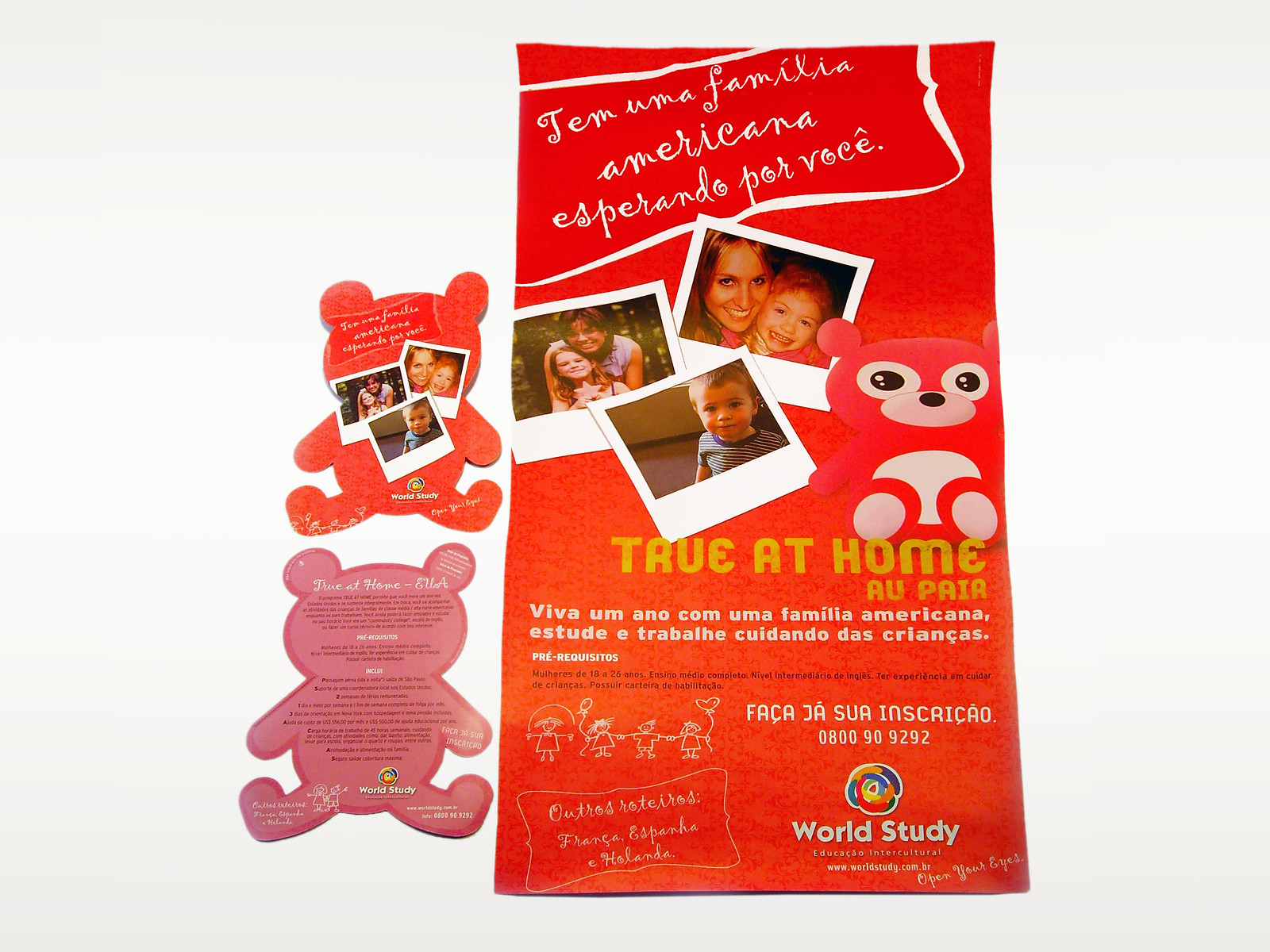This vibrant postcard, predominantly featuring red and pink tones, depicts a joyful gathering of families and children, all smiling warmly at the camera. The lively and colorful image suggests a celebration of family and togetherness, possibly hinting at themes of adoption or community bonding. Adding to its unique charm are the illustrations of red and pink bears, which harmonize with the main color scheme. The text on the postcard is written in French, adding an additional layer of intrigue for those not fluent in the language.